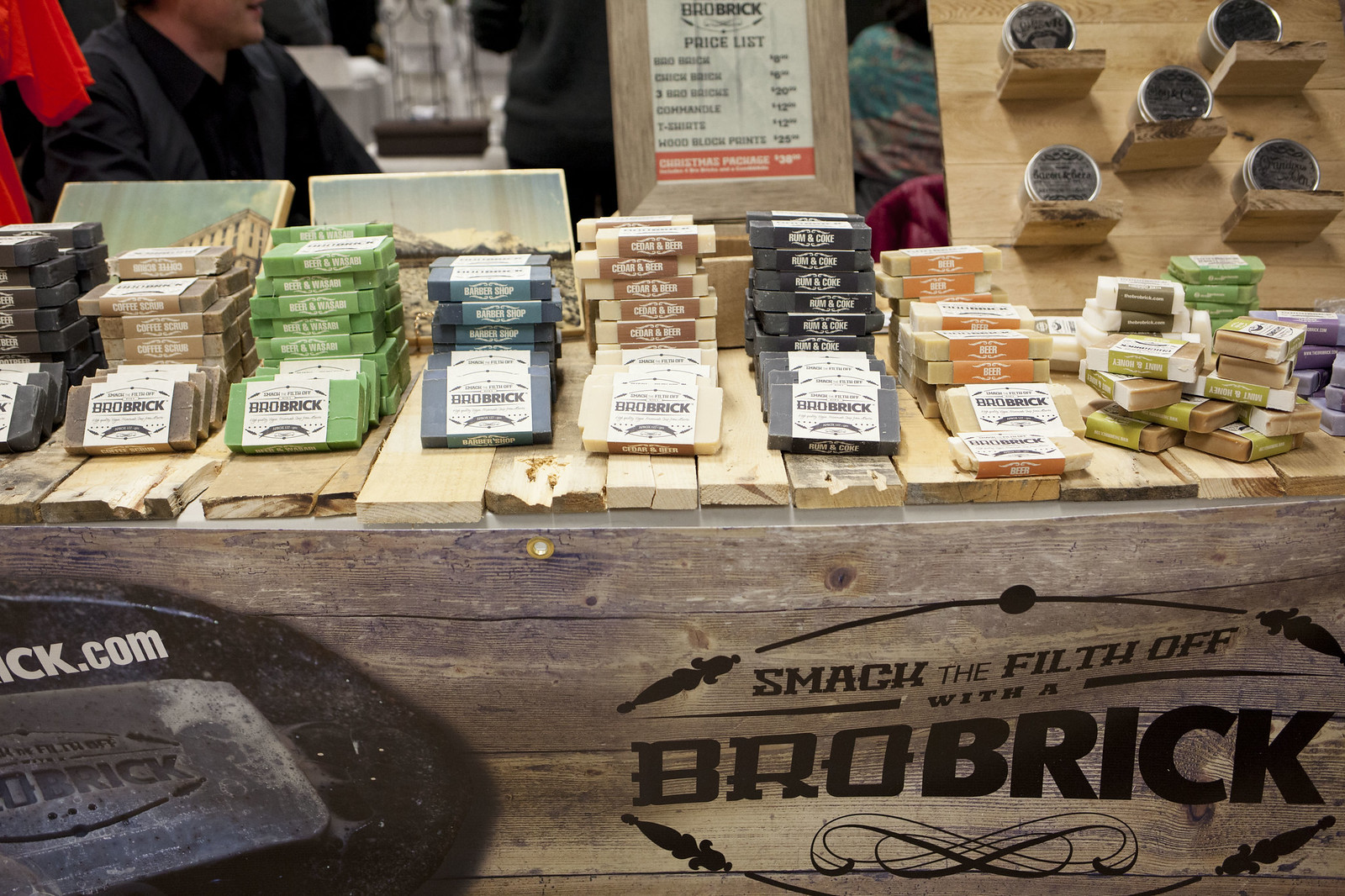The image showcases a rustic wooden table made of rough, horizontally-laid planks, prominently displaying a variety of homemade soap bars under the brand "Bro Brick." In front of the table is a fake wooden sign inscribed with "Smack the filth off with a Bro Brick." The soaps come in an array of vibrant colors including green, navy blue, white, dark brown, light blue, orange, and lime green, each wrapped with labels bearing the Bro Brick logo. Toward the back right of the table, a piece of wood is propped up, holding more products that include silver containers with black labels, possibly additional toiletry items. To the left, another wooden prop displays a pricelist, though the details are not legible. Stacks of these colorful soap bars and possible additional grooming items create a visually appealing, bustling shop display.